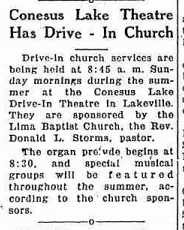This image depicts a small clipping from an old newspaper, characterized by its distinct vintage font and white background. The clipping's modest size suggests it is from a classified section, complete with visible boundary lines on the top, right, and bottom edges, indicating it was clipped from a full page. At the top of this single-paragraph article, the bold title reads, "Conesus Lake Theater Has Drive-In Church." Below this title, in regular font, the text announces that drive-in church services are being held at 8:45 a.m. on Sunday mornings during the summer at the Conesus Lake Drive-In Theater in Lakeville. These services are organized by the Lima Baptist Church, with the Reverend Donald L. Storms serving as pastor. An organ prelude starts at 8:30, and various special musical groups will perform throughout the summer, as noted by the church sponsors. Additionally, the clipping suggests that a portion of the original column may have been cut off, as indicated by partially visible letters on the right side.